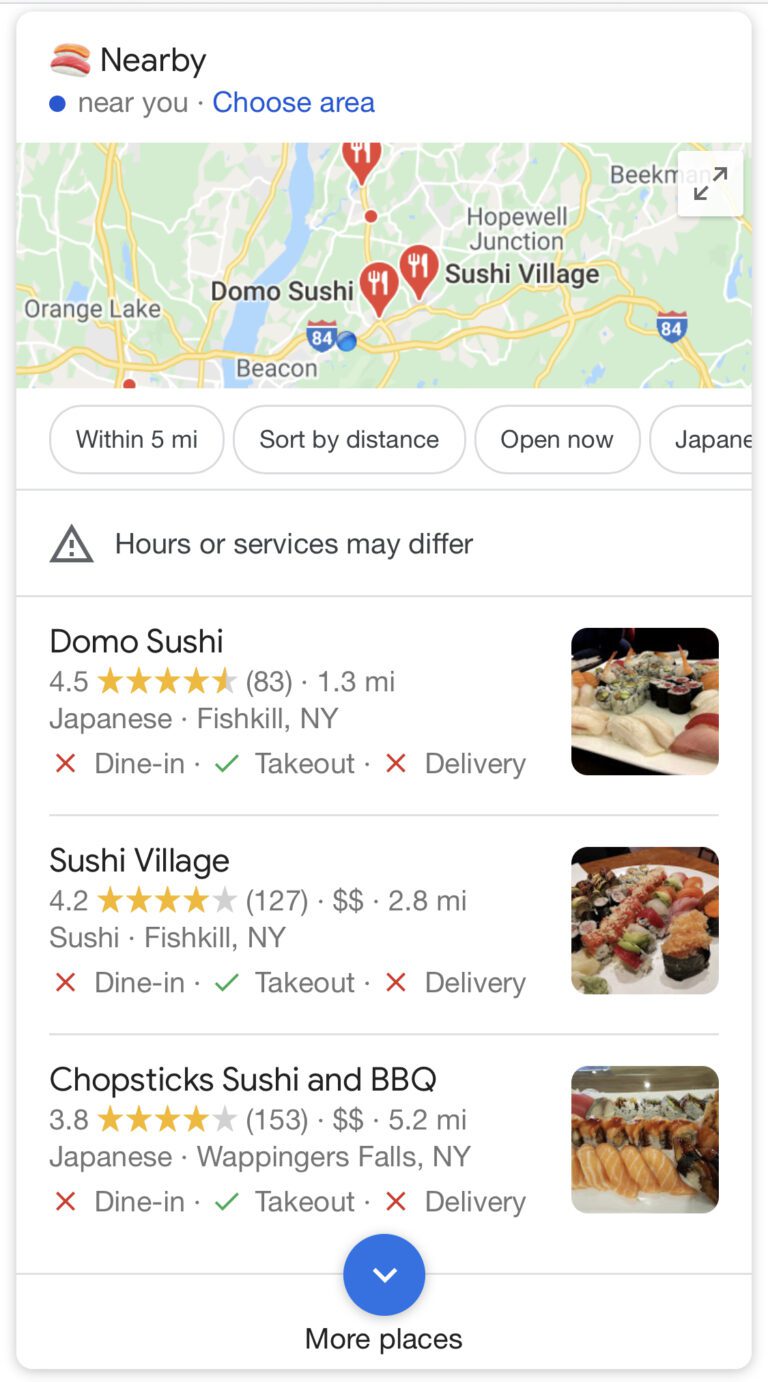The image features a screenshot of the Google Maps interface. At the top, the screen displays tabs titled "Nearby," "Near You," and, in blue text, "Choose Area." Below these options is the map displaying an area with a predominantly green landscape, intersected by yellow lines representing highways and a river running vertically through the center. Three dark red icons indicate the locations of restaurants.

Further down, a section provides various filters and categories: "Within 5 miles," "Sort by Distance," "Open Now," and "Japanese," underlined by the note "Hours or services may differ."

The first restaurant listing is "Domo Sushi," with a rating of 4.5 stars based on 83 reviews. It is located 1.3 miles away and categorized under Japanese cuisine in Fishkill, New York. An image of the restaurant is positioned to the right.

The second listing is "Sushi Village," rated 4.2 stars from 127 reviews, situated 2.8 miles away in Fishkill, New York. There is an adjacent image portraying the restaurant's food.

The third restaurant is "Chopsticks Sushi & BBQ," with a 3.8-star rating and 153 reviews. It is 5.2 miles away, located in Wappingers Falls, New York. This listing also has a corresponding image to the right.

At the very bottom of the screen, there is a blue circle with a downward-pointing arrow, and beneath it, the text "More places" is displayed in black.